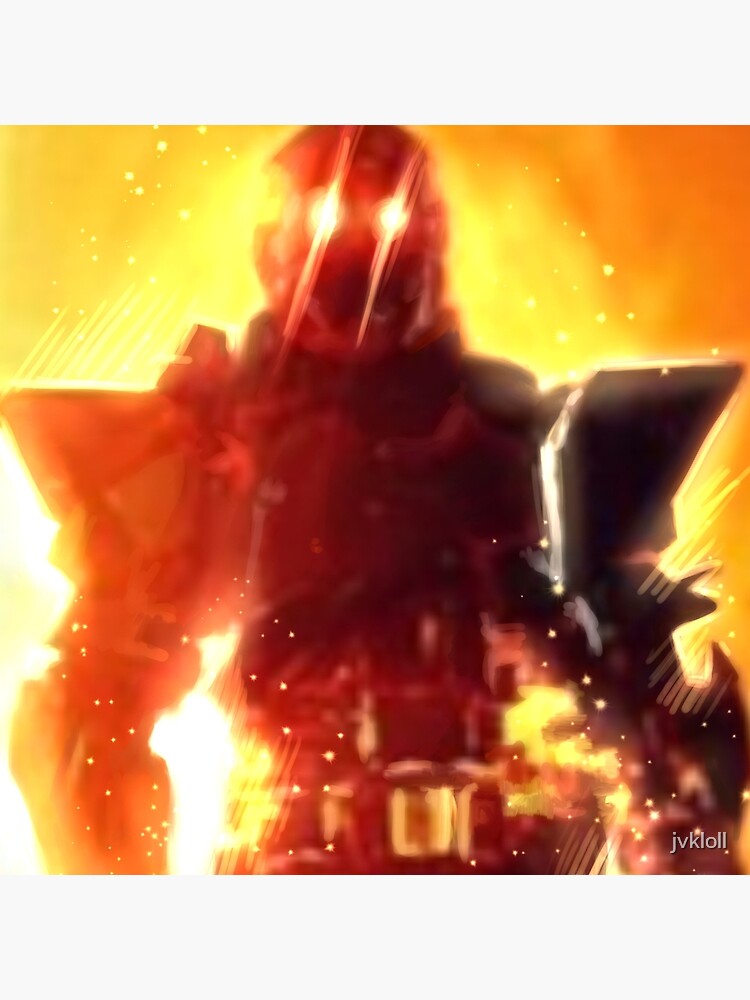This image features a vividly depicted robotic figure, centrally positioned with glowing yellow eyes that exude an eerie, supernatural aura. The figure is heavily armored, reminiscent of a superhero, and has a striking gold belt buckle. Surrounding the robotic entity’s head are specks of yellow light, resembling embers or fiery sparks, which intensify the dramatic atmosphere. In the background, a bright yellow and orange explosion-like blast adds to the dynamic composition. The text "JVKLOLL" appears in light gray lowercase letters, positioned directly over the figure’s torso. This artwork, with its crisp, bold colors and intense imagery, evokes the style of modern action video games like Doom.